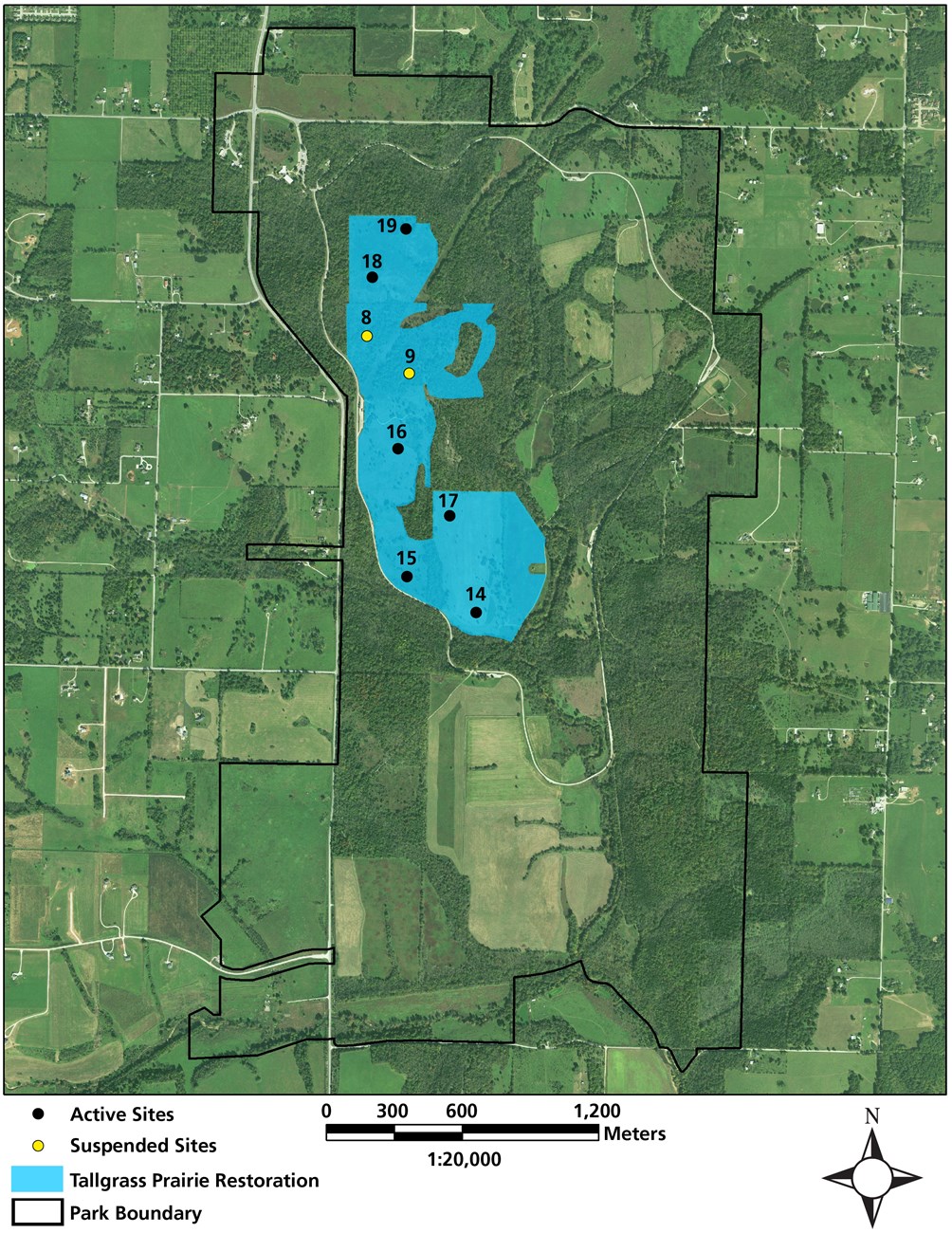This image displays a detailed aerial map dominated by various shades of green, indicating different sections of a landscape. A prominent blue lake occupies the center, housing several black and yellow dots which correspond to different sites. Surrounding the landscape are white-bordered sections, likely denoting parcels of land. 

At the bottom of the map is a black and white legend including:
- A black dot labeled "Active Sites"
- A yellow dot labeled "Suspended Sites"
- A blue bar marked "Tall Grass Prairie Restoration"
- A white rectangle outlined in black for "Park Boundary"

Adjacent to the legend is a scale bar with numbers 0, 300, 600, and 1200, representing meters. Below the scale, there is a notation "1,20,000". 

A compass located in the bottom right corner indicates the cardinal directions, with 'N' labeled at the top for north.